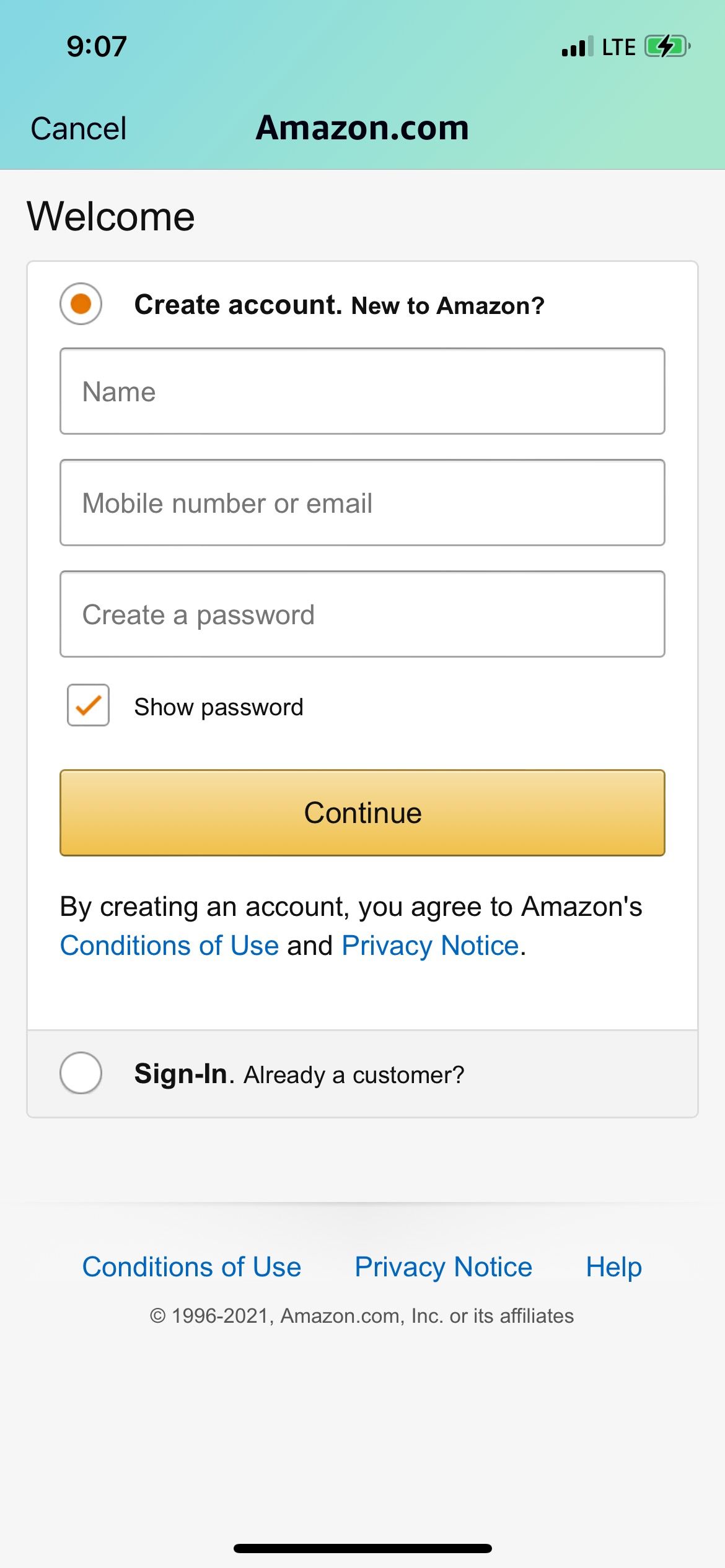The image shows the user interface of a mobile device displaying Amazon's account creation screen. At the top, a status bar features a gradient rectangle transitioning from bluish-green on the right to a lighter green on the left. The top left corner displays the time, "9:07," while to the right, four signal bars gradually increase in size, with three in black and one in dark green, beside the label "LTE." A battery icon with a crooked "Z" symbol is also visible.

Below the status bar, the screen is layered with various sections. The left corner features a "Cancel" option, and centrally aligned text reads "Amazon.com." Directly underneath is a gray rectangle with the word "Welcome," containing a white inner rectangle. This inner rectangle displays a gray-outlined circle with an orange center, accompanied by the text "Create Account."

The lower part of the screen includes fields outlined in gray for "Name," "Mobile Number or Email," and "Create Password." Adjacent to the password field is a gray-outlined square with a yellow checkmark, labeled "Show Password." An orange rectangle, outlined in black with the text "Continue," lies beneath these fields.

The terms of service are mentioned below, stating: "By creating an account you agree to Amazon's," followed by a blue hyperlink, "Conditions of Use," and then "and" in black, with another blue hyperlink, "Privacy Notice." At the very bottom, there's a small white circle outlined in black with the text "Sign In," next to "Already a customer?" and another series of blue hyperlinks: "Conditions of Use," "Privacy Notice," and "Help." The remaining text is small and unclear, and a black bar runs along the bottom edge of the screen.